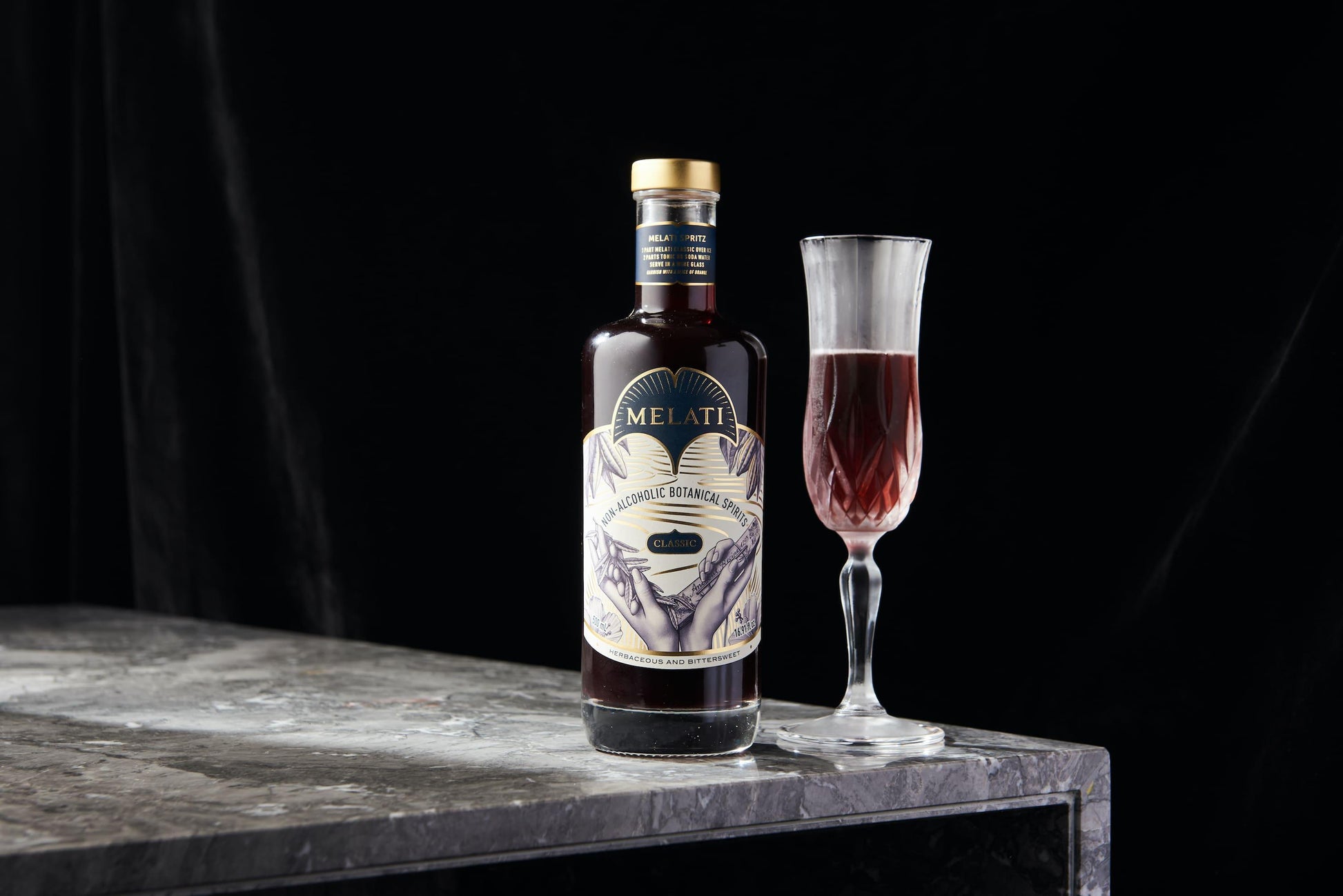Set against a velvety black drape, this studio-stylized product photo features a bottle of Malati, a non-alcoholic botanical spirit with a classic, herbaceous, and bittersweet flavor. The bottle, adorned with an etched gold label and capped with a gold top, stands on a gray marble countertop. The label prominently displays the brand name "Malati" and the phrase "non-alcoholic botanical spirits." The intricate artwork on the label includes black and white illustrations of hands, herbs, and a box. Beside the bottle sits a sleek, long-stemmed martini glass, filled halfway with a dark red liquid, adding a touch of elegance to the composition.